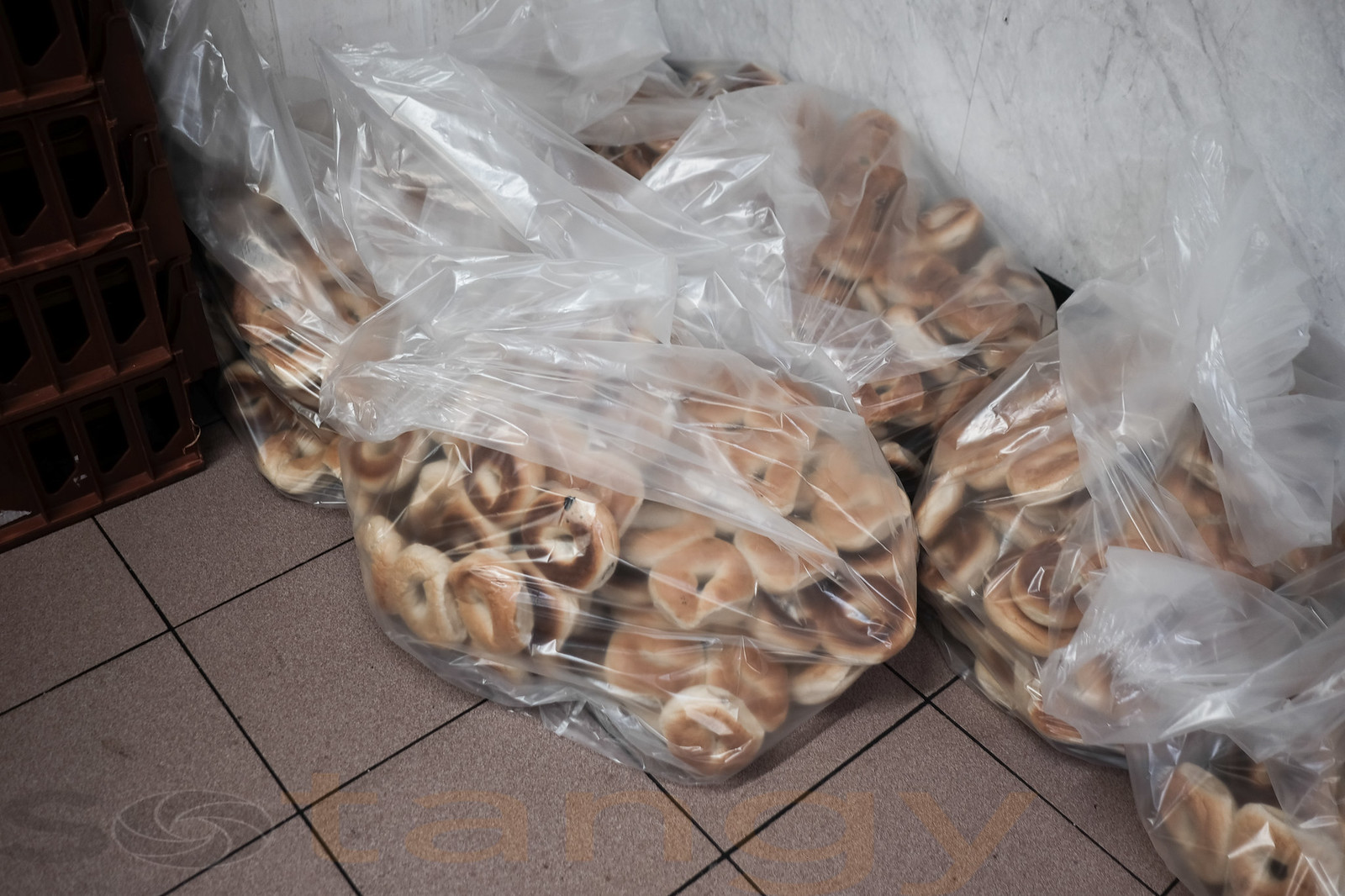This color photograph depicts six large, heavy-duty, clear plastic bags filled with toasted bagels, likely from a bakery. The bags are placed in the corner of a room. The flooring is dark gray speckled industrial tile with black grout, and a faint, wide watermark stretches across the bottom left corner of the image, displaying the letters "S-O-T-A-N-G-Y" with an "O" resembling a camera shutter. The wall visible at the top right is a white-gray marble pattern. The photograph is devoid of people, animals, or other distinguishable objects, emphasizing the abundant bags of bagels against the stark interior setting.